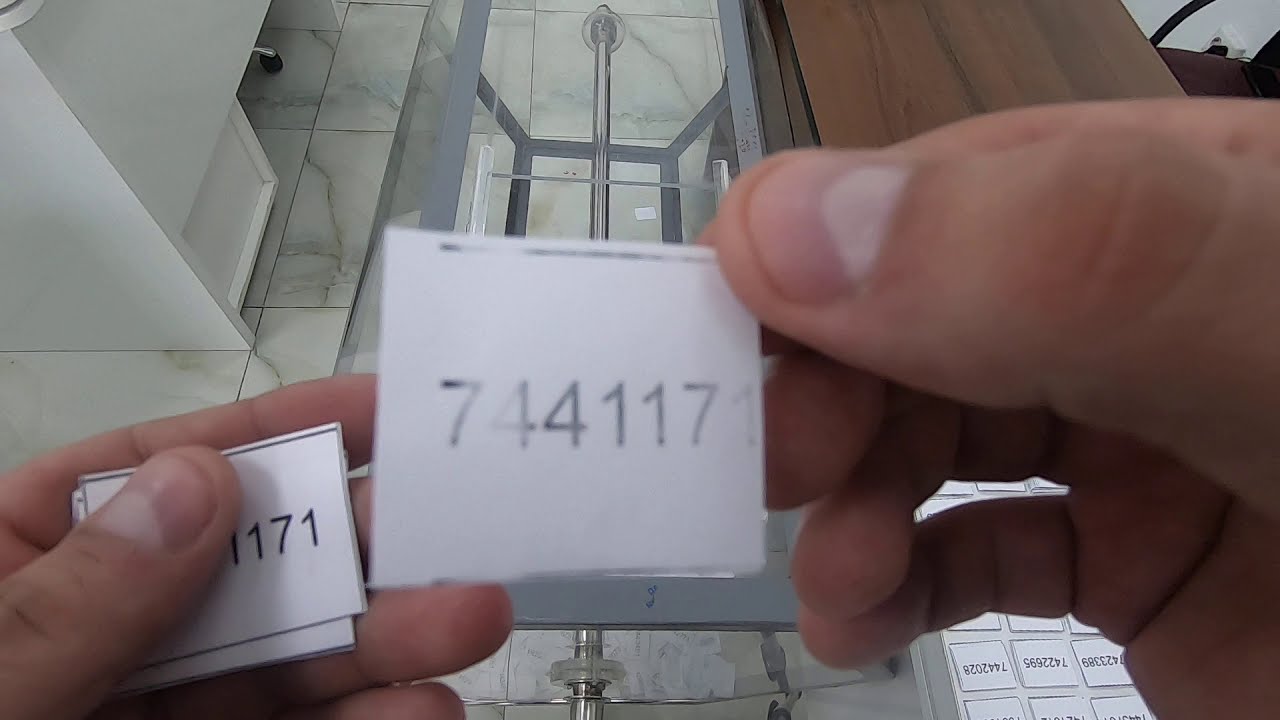In the image, a person is holding various white paper squares marked with numbers. In their right hand, they are holding a square with the black-inked number 7441171. Their left hand is slightly below and holds multiple squares, with the topmost showing the last four digits "1171" partially obscured by their thumb. Directly in front of them is a glass or acrylic container framed with gray metal and equipped with a rolling handle. To the immediate bottom right behind the person's right hand lie additional numbered paper squares. The right side of the image features a wooden tabletop with a vertical wood grain pattern interspersed with darker lines. The left side includes a white desk, and the white marble tile floor completes the scene.